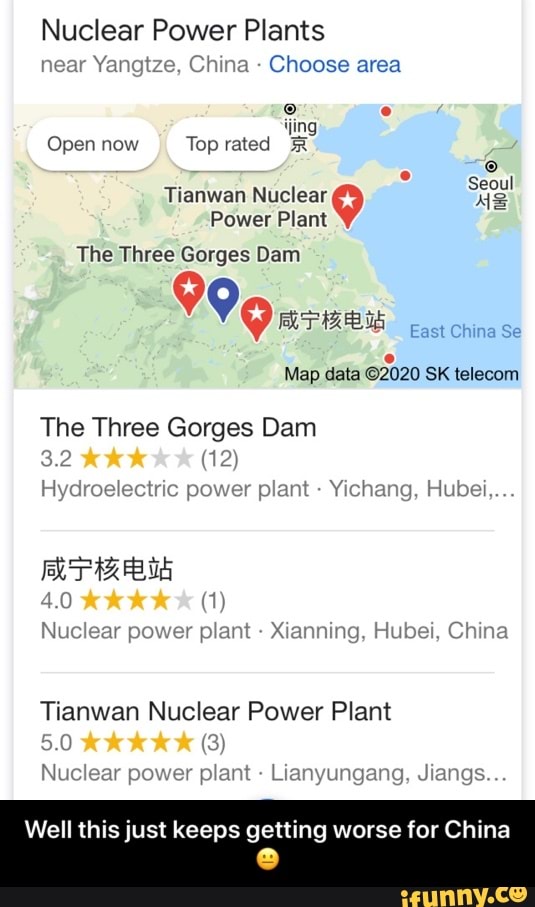The image displays search results on Google Maps for "Nuclear Power Plants Near Yangtze, China." At the top, there is a prominent rectangular area with a white background. The heading "Nuclear Power Plants" is displayed in a semi-rounded sans-serif font in black, with a smaller grey subheading that reads "Near Yangtze, China." A grey bullet point separates this from a blue, clickable "Choose Area" link.

The map itself is marked with three red pins featuring white stars and a white border, and one dark blue pin with a white circle and border. In the top left corner, two white oval overlays indicate options, reading "Open Now" on the left and "Top Rated" on the right.

In the bottom right corner, "map data ©2020 SK telecom" is written in small black sans-serif font. Below the map, the first listing is for "The Three Gorges Dam." It appears in black text, with a grey subtext denoting a rating of "3.2". This rating is visually represented by three filled yellow-orange stars out of five, with the remaining two being light grey. Accompanying this are grey parentheses indicating "12 reviews" in a smaller font.